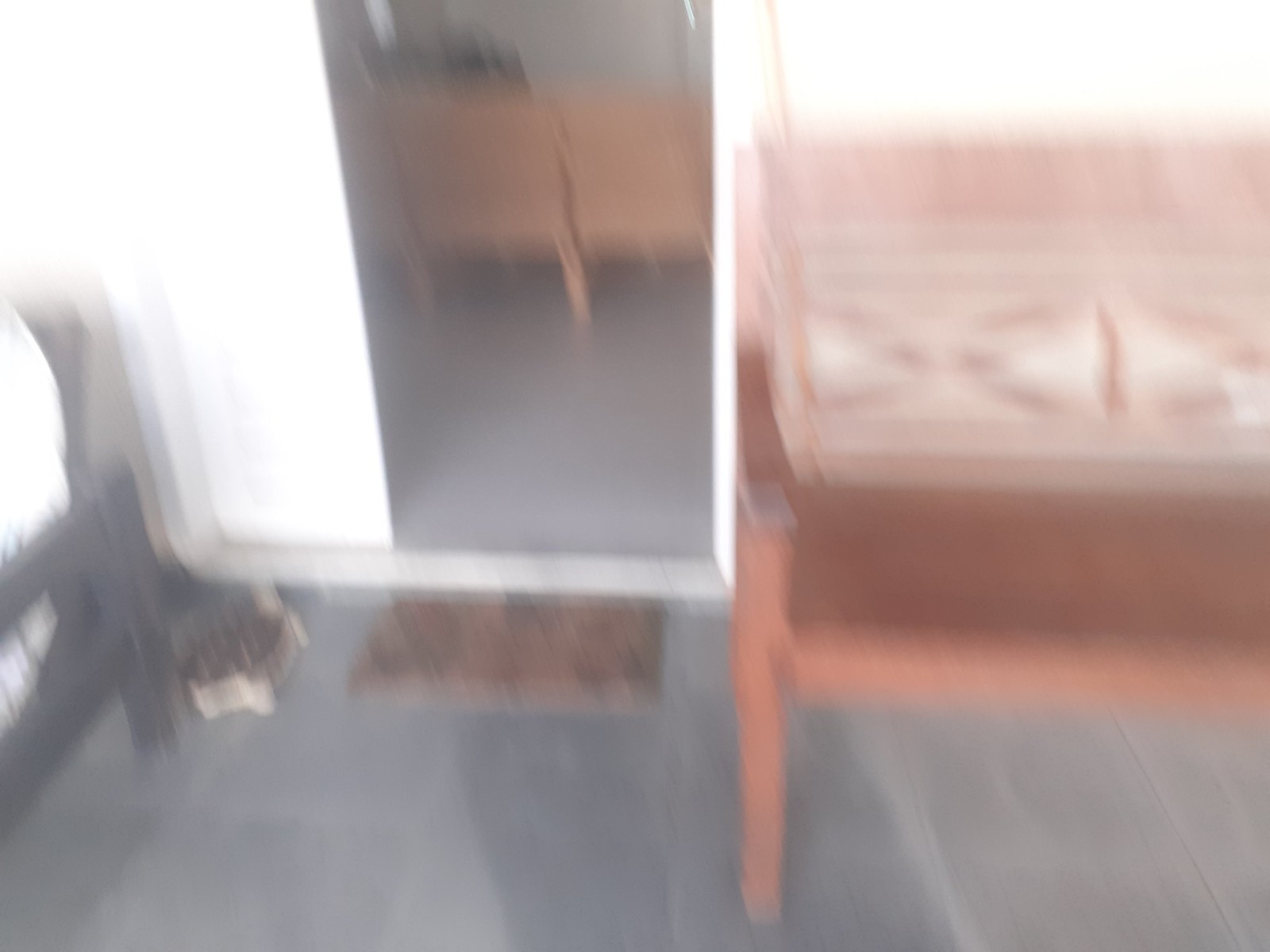A blurred image depicts an interior setting with various elements discernible despite the lack of clarity. On the right side, a structure resembling a bench or table can be identified by its visible leg. The seating area towards the back features white upholstery accented with brown wooden hatches. The floor appears to be covered with dark-colored tiles, possibly black or gray, contributing to the image's overall brightness, which seems overly enhanced.

A brown welcome mat is positioned in front of a doorway, suggesting an entry point into another space. Additionally, a brown table is visible, adding to the room's furnishing. On the left side, there's an indistinct black object, and at the bottom left, a pet feeder is present, indicating the room's multifunctional nature.